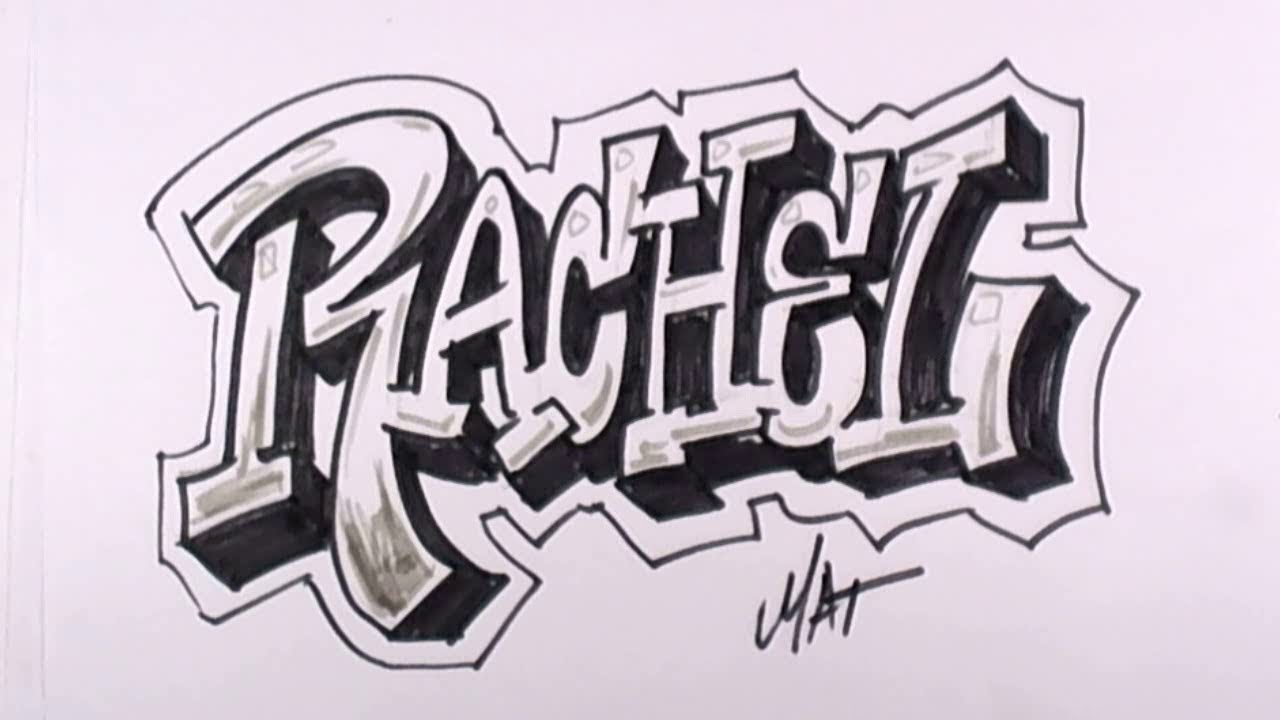The image depicts a graffiti-style artwork of the name "Rachel," rendered on white paper. The letters are blocky and three-dimensional, reminiscent of 1980s bubbly graffiti, with a stark black outline and additional gray shading to enhance the 3D effect. The artist's signature, "Matt" (spelled M-A-T), is located in the lower right-hand corner, just beneath the prominent "Rachel" tag. The monochromatic black and gray design bears a polished finish, similar to that of tourist illustrations or personalized name plates, albeit with a distinct graffiti flair.